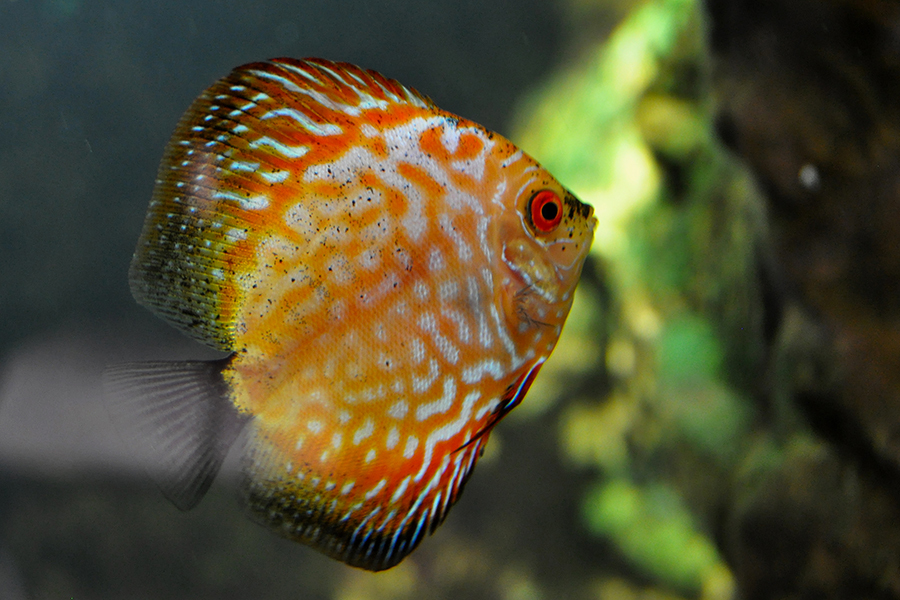This highly detailed, full-color photograph features a tropical, heart-shaped fish, predominantly orange with intricate vein-like patterns and black specks across its body. The fish, centered slightly to the left, is captured in stunning high resolution, showcasing its vivid red eyes with black pupils and black dots around its nose and mouth. The fish's upper and lower fins exhibit a blend of blue and red hues, while its tail fin is transparent and gray. The background is mostly out-of-focus dark tones with hints of green, suggesting aquatic plants, and some rock formations, creating a striking contrast that highlights the vibrant details of the fish.